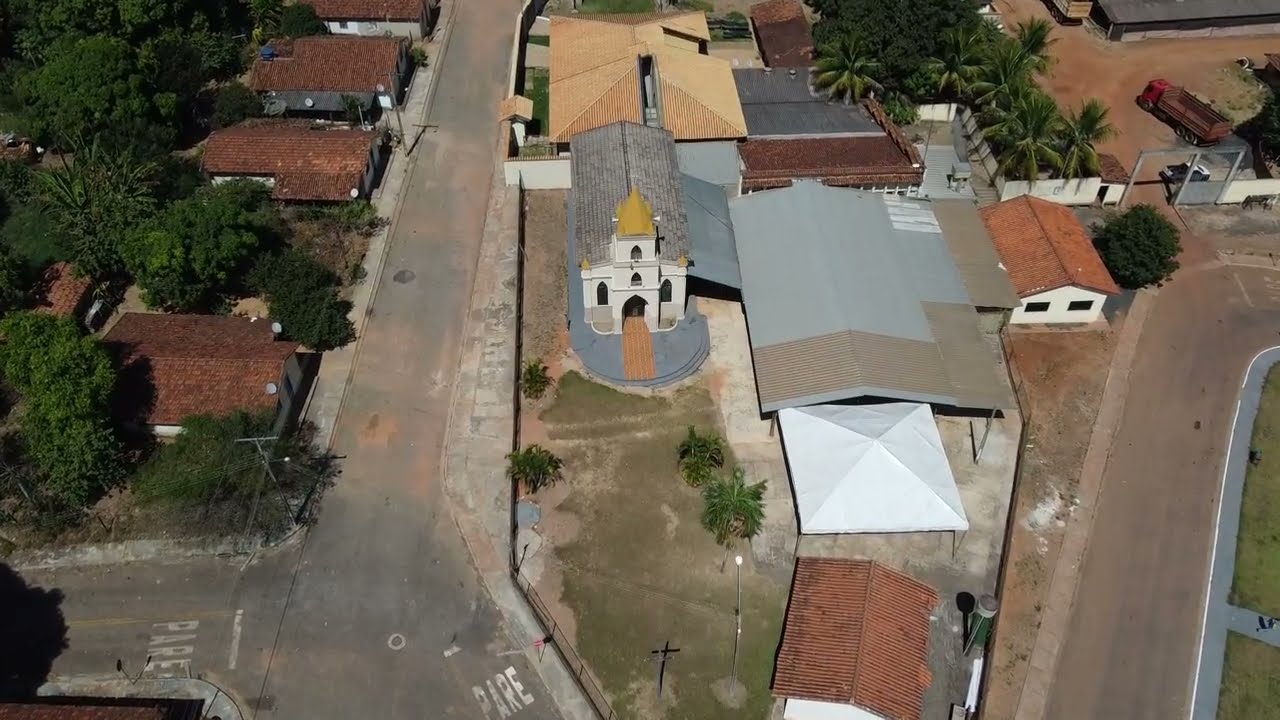This aerial photograph showcases a bustling street scene dominated by a picturesque church with a white facade, gray roof, and a prominent golden spire. The church, surrounded by a large greenish-brown field dotted with several bright green trees and a distinct black cross near the bottom of the frame, serves as the image’s focal point. Adjacent to the church are various buildings, primarily featuring red and brown roofs, alongside some that are gray, blue, and white. Notably, a building behind the church sports a striking gold roof. 

Two streets are visible in the image: one descends from the right-hand side, making a turn at the bottom, while the other stretches from the top to bottom, splitting into two—one segment veering left and another continuing straight. The roads are light gray with lighter gray sidewalks. Red dirt paths intersperse these buildings, supplanted by lush dark green trees of diverse species. 

On the left side of the church is another road flanked by buildings—potentially houses—enshrouded by trees. To the right, a secondary road meanders into the background. An array of rectangular, single-story buildings with brown roofs occupies the bottom right. Amid these structures, a large flat-roofed building and another with a prominent vertical, light brown roof are observable. 

In the middle-left section, adjacent to the church, there is an open area with a big roof covering but no building beneath it. Highlighting the surrounding details, a car behind a fence and a red truck parked in a distant lot underscore the everyday life interlaid with the serene setting. Palm trees punctuate the background, enriching the exotic ambiance of this vibrant neighborhood scene.